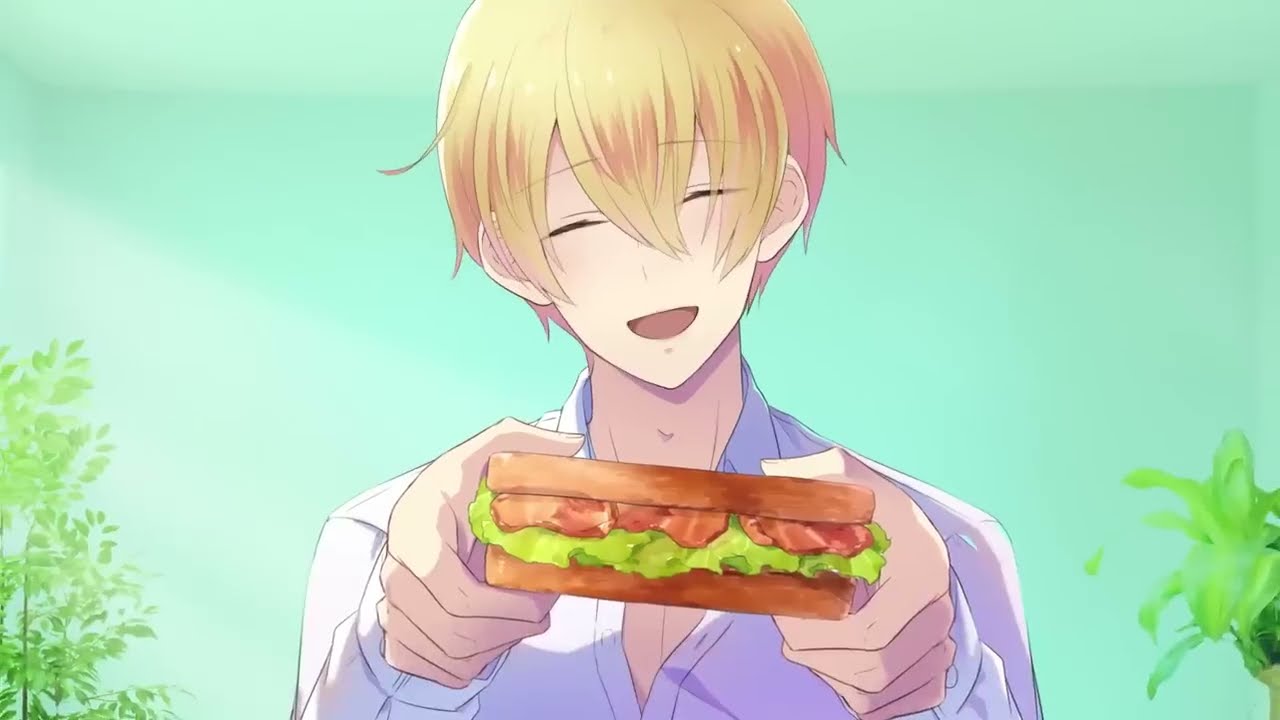This anime-inspired illustration features a young, blonde boy with fair skin, characterized by his dramatically extended bangs that obscure his nose. With his eyes closed and a wide, joyful smile revealing his pointed chin, he eagerly extends a sandwich towards the viewer. The sandwich, constructed of two slices of bread, includes visible layers of greenery, perhaps lettuce, and several pieces of meat, likely bacon, suggesting it might be a BLT. He wears a white button-up shirt with the top two or three buttons undone, emphasizing his casual, carefree demeanor. The background depicts a sunny day with a light greenish-blue sky and a couple of trees positioned at the lower left and right corners, akin to a serene park setting. The overall scene radiates happiness and the inviting gesture suggests he is offering the sandwich to someone, creating a warm, engaging moment captured with a touch of anime-style artistry reminiscent of Dragon Ball Z.